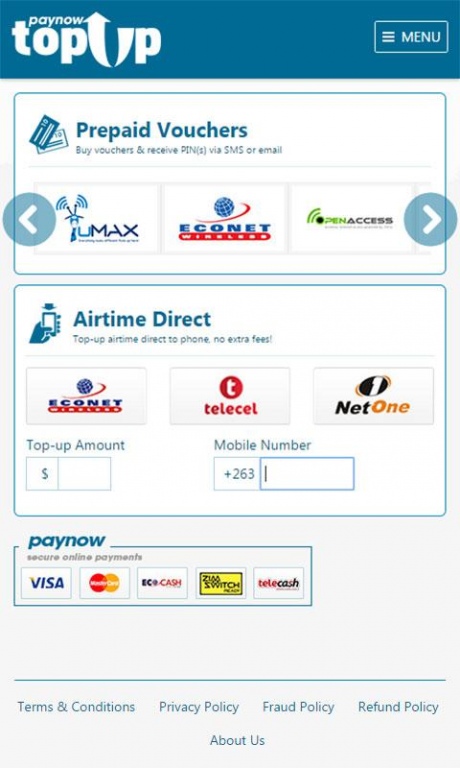The image showcases a mobile app interface designed for topping up prepaid cell phone plans. At the top, a blue horizontal bar spans across the screen, displaying options such as "Pay Now" and "Top-Up." In the top right corner, a menu button is present.

Below this bar, there are two rectangular sections outlined in blue. The first section is labeled "Prepaid Vouchers" and includes options to buy vouchers and receive PINs via SMS or email. Within this section, vouchers are available for various providers such as Umax, Econet, Open Access, and Airtime Direct.

The second section, labeled "Top-Up Airtime Direct," offers a service to top up airtime directly to a phone without extra fees. Providers for this service include Econet, Telecel, and NetOne. Users have the option to add the top-up amount and enter the phone number they wish to credit.

At the bottom of the screen, there is a "Pay Now" button, along with icons representing secure online payment options including Visa, MasterCard, EcoCash, ZimSwitch, and Telecash.